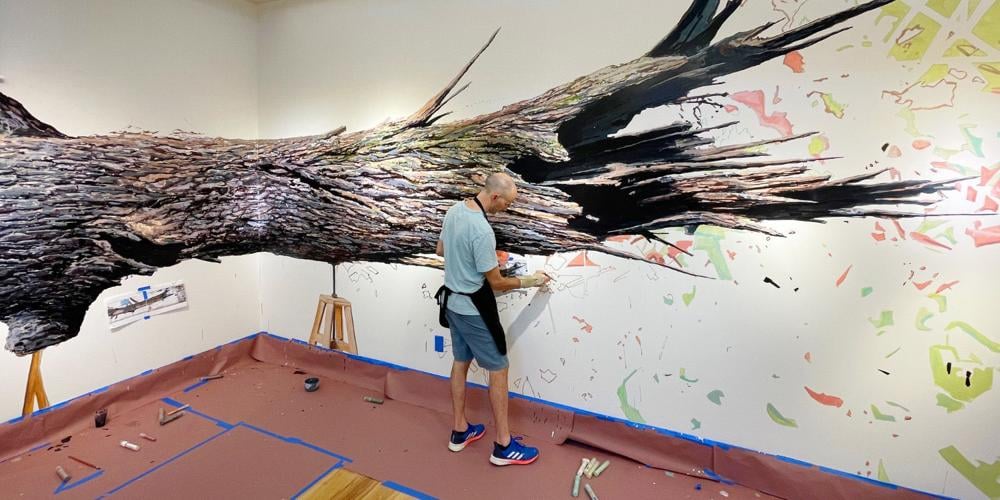In the image, a white, bald man is painting a mural in the bright corner of a large room. The horizontal, rectangular picture showcases him standing where two white walls meet. The floor is protected with a dark pink tarp securely taped with blue painter's tape. The mural features a large tree trunk, painted with a mixture of browns and grays, starting wide on the left wall, narrowing as it wraps around the corner to the right wall. The man is working on the right wall, adding intricate details where the trunk appears broken off, with sharp, thin lines extending upwards. He is dressed in a light blue t-shirt, blue shorts, and blue sneakers, complemented by a black apron and white gloves. He appears to be holding a paintbrush and wears glasses, adding detailed symbols and shapes below the tree trunk, incorporating red and green splashes of color that resemble multicolored snowflakes or pieces yet to be completed. The well-lit setting ensures that every detail of his artistic process is clearly visible.